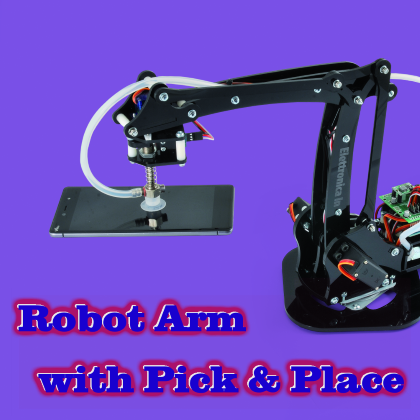The image depicts a compact black robot arm designed for pick and place operations, set against a vivid purple background. The arm emerges from a sturdy base, rises vertically, and extends horizontally at a 90-degree angle. Throughout its structure, the robot arm features various rivets and silver screws, facilitating its jointed movements. Red wires and a green circuit board are visible at the base, suggesting an intricate electronic setup. Additionally, a white tube, possibly part of a hydraulic system, is integrated into the arm's mechanism. Attached to the end of the arm is a metal plate, which the robot may use to pick up or place items. The picture is captioned "Robot Arm with Pick & Place" at the bottom.